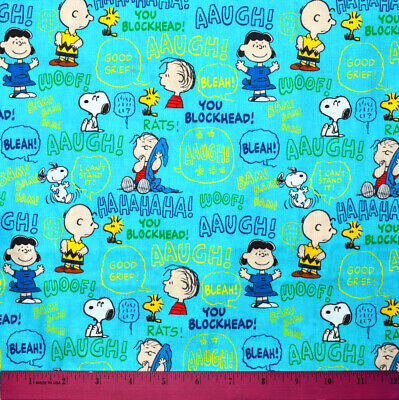This vibrant image features a repeating pattern of characters from the Peanuts cartoons against a bright turquoise background, potentially designed as wrapping paper or a decorative poster. Prominent characters include Charlie Brown in his classic yellow shirt with a black zigzag, red shoes, and black pants. Close by is his sister Sally, dressed in a blue dress. Snoopy, the white dog with black ears, black nose, and black eyes, also appears sporadically, sometimes with Linus below him carrying his blue blanket and sucking his thumb. Linus is sometimes seen in his red and black striped shirt. Lucy, with her short black hair, appears as well, dressed in a blue dress with white shoes and blue socks. Woodstock, the little yellow bird, is present in the scene, adding to the cheerful dynamic.

Accompanying the characters are various phrases from the comic strip in text colors of blue, green, and yellow, including "ha ha ha ha," "AAUGH!," "you blockhead," "rats," "bleah," and "good grief," adding a playful touch. A purple ruler measuring exactly 12 inches can be seen at the bottom of the image, giving a sense of scale to this detailed pattern. The repetitive design and lively color scheme suggest it could be used for wrapping paper, wallpaper, or any other decorative purpose.